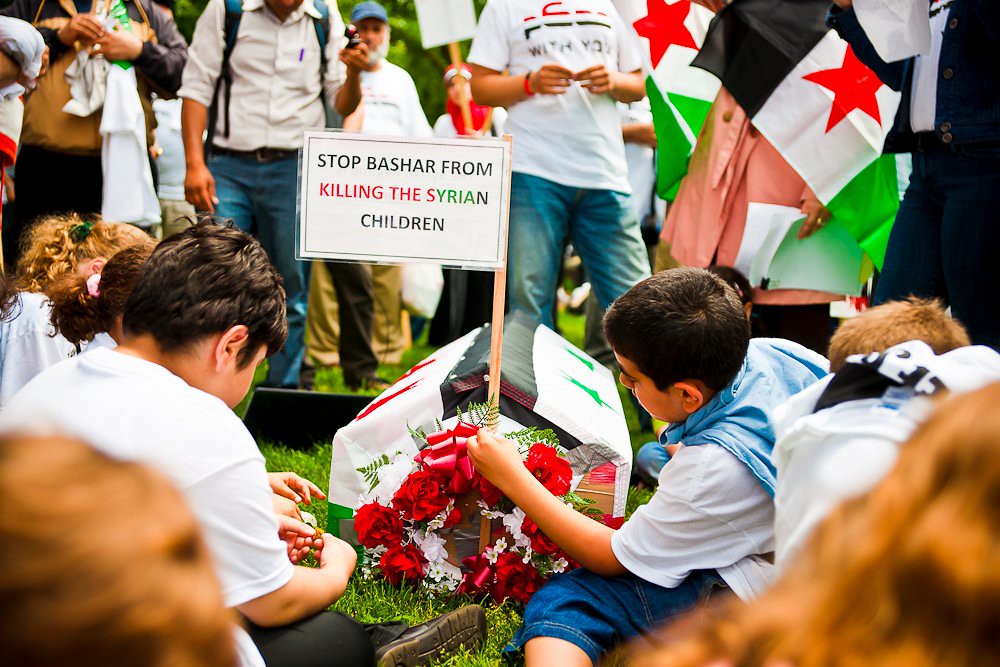In a vibrant and poignant scene at a cemetery, a somber gathering unfolds as both children and adults come together in a peaceful protest. Central to the image is a small coffin draped with the Syrian flag, featuring red stars on a white background with black and green stripes. In front of the coffin lies a wreath of red and white roses intertwined with green leaves. A child in the forefront stands out, dressed in jean shorts, a white t-shirt, and a blue shirt tied around his neck, holding a sign that reads, "Stop Bashar from killing the Syrian children." Beside him, another child in a white shirt and black pants sits on the green grass.

Surrounding the scene, adults and children alike, some seated and others standing with their heads partially out of the frame, hold flags identical to the one on the coffin. The flags prominently display red stars against a backdrop of black, white, and green stripes. The vibrant green lawn underscores the sharp visual of the photograph, capturing the stark contrast between the serenity of the landscape and the gravity of the protest's message.